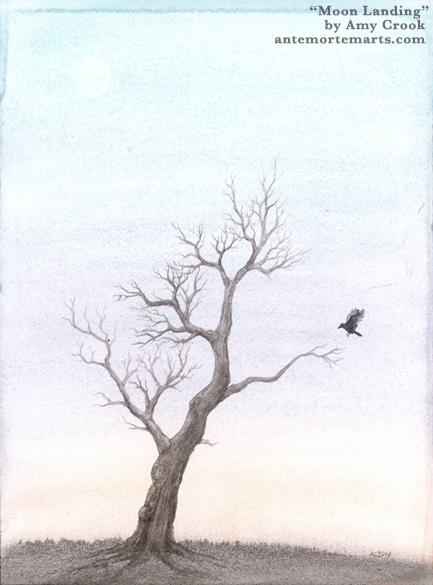The image, titled "Moon Landing" by Amy Crook and hosted on TameArts.com, is a finely detailed pencil sketch in portrait orientation. It depicts a barren, dead tree as the central subject, occupying slightly more than half the height of the artwork. The tree's trunk is wide at the base, curves gently to the right, and branches out in multiple directions, revealing its leafless, skeletal structure. The backdrop presents a serene, clear sky rendered in subtle gradients from light blue at the top to touches of light purple and orange near the horizon, suggesting a tranquil daylight setting.

In the foreground, the ground is shaded in grey and beige tones, mimicking a grassy field. The sky is clear, emphasizing the stark solitude of the tree. A black bird, likely a crow, is captured in profile with its wings spread wide, poised to land on a branch on the tree's right side. This dynamic moment heightens the atmospheric eeriness of the scene.

Adding to the image's intrigue, there is text in dark gray located at the top right corner. It reads, “Moon Landing” in quotation marks, followed by “by Amy Crook” and “TameArts.com." The artwork collectively evokes a sense of somber beauty and stillness, characteristic of pencil sketch artistry.